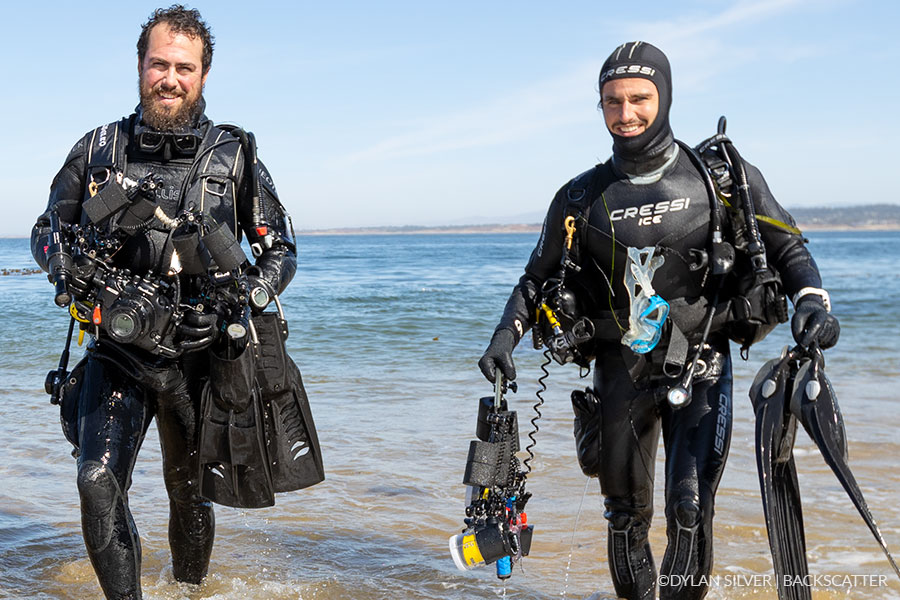In the image, two tan scuba divers are wading through ankle-deep water, heading towards the shore. The diver on the left has his hood off, while the one on the right still wears his hood. Both divers are dressed entirely in black wetsuits and carry an array of equipment, including swim fins and what appears to be camera gear, suggesting they might be filming an underwater documentary. They are smiling and appear well-prepared for their dive. The ocean behind them transitions from blue to a brownish hue near the shore, with gentle waves rippling the surface. The background reveals a hilly shoreline under a predominantly blue sky with very faint clouds. On the diver's black long-sleeve shirt, the brand "Cressy" is visible. In the bottom right corner of the image, "Copyright Dylan Silver" is marked in white font.